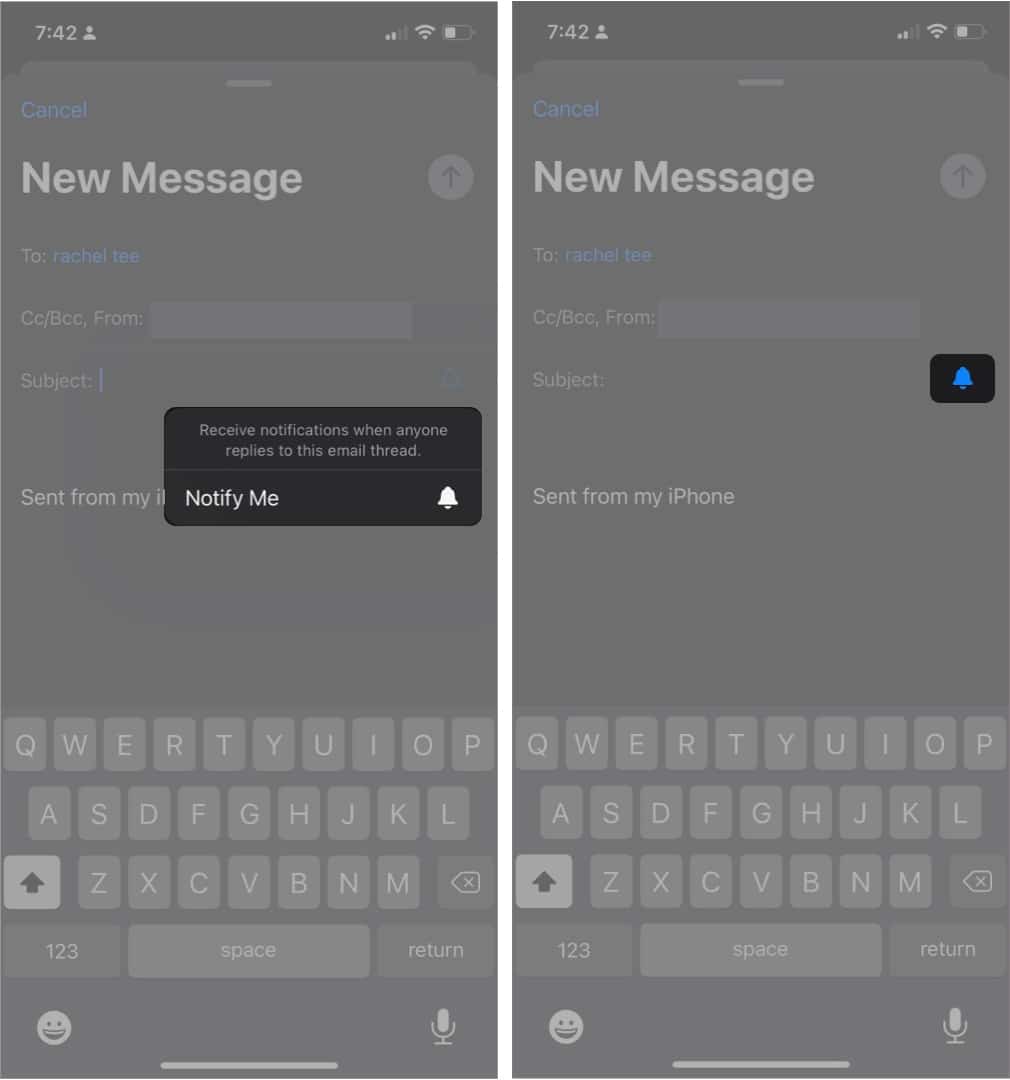The image consists of two side-by-side screenshots, most likely taken from an iPhone. Both screenshots showcase an identical view of an email composition screen, with minor variations between them. 

In both screenshots, the top status bar displays the time "7:42" on the left, along with the Wi-Fi, signal strength, and battery icons on the right. Below the status bar, the screen shows standard email composition fields, including a blue "Cancel" button on the upper left, and "New Message" with the recipient "To: Rachel TEE." 

Directly below the recipient field, there is a "Cc/Bcc" line and a "Subject" line, followed by the text "Sent from my iPhone." At the bottom of each screenshot, the on-screen keyboard is visible, complete with a happy face emoji icon on the left, a microphone symbol on the right, and various alphabet keys.

The primary difference between the two screenshots lies in the email body area:
- The left screenshot features a semi-transparent black box with text that reads, "Receive notifications when anyone replies to this email thread," accompanied by a small bell icon and a "Notify Me" button.
- In contrast, the right screenshot has only a blue bell icon to the right of the subject line.

Overall, the image depicts the subtle differences in user notification options within an iPhone email interface.